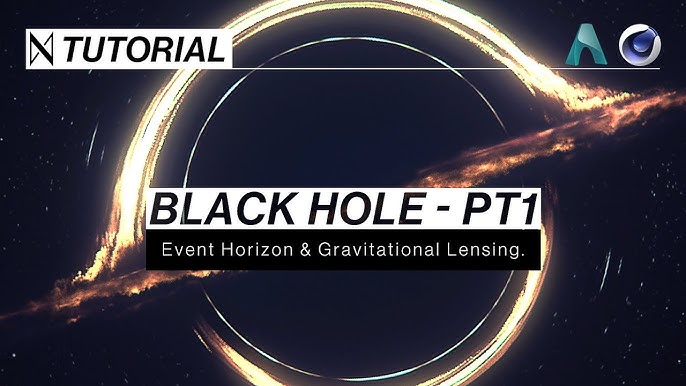This image appears to be a detailed tutorial thumbnail on creating a visual representation of a black hole, drawing inspiration from the movie "Interstellar." Dominating the center of the image is a large circular black hole that occupies the full vertical span. The innermost part of this black hole is pure black, symbolizing the event horizon. Encircling it is a deep, bright yellow ring with a thinner, equally bright yellow line towards the inside edge, giving it a fiery, almost incandescent appearance. 

A striking feature of this black hole is an orange streak of light that diagonally traverses from the upper right to the lower left, cutting through both the black core and the vibrant amber circumference, creating a dramatic contrast. The background on either side of the black hole is pitch black, peppered with white stars that spiral and appear stretched as if distorted by the gravitational lensing effect of the black hole. 

In the upper left corner, there is a white rectangular box with bold black text that reads "TUTORIAL." A horizontal line extends from the rectangle, intersecting with a small teal 3D 'A' and a white sphere with a blue center, adding a touch of modern graphic elements. Central to the image, another white rectangle contains the text "Black Hole - Part 1," and directly beneath it, a black rectangle displays the subtitle "Event Horizon and Gravitational Lensing" in smaller white text.